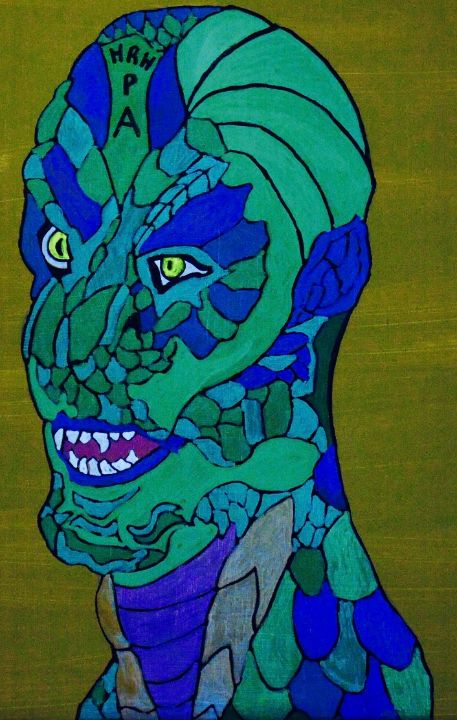This detailed and vibrant painting showcases a fictitious creature that appears to be a hybrid of man and beast. Dominating the olive green canvas, the face and upper body of this monster-like figure are meticulously depicted. The creature's head is vivid green with a pronounced scalp, and its piercing lime green eyes are striking. It has an open mouth bordered with shades of blue and purple, revealing sharp, fanged teeth above and below. The forehead prominently displays the letters "MRWPA," flanked by bluish-purple hues that extend to the area around its ears.

The beast's neck, reminiscent of lizard skin, is decorated with patterns resembling oblong stones or scales, colored in various shades of blues, greens, and turquoises that continue down to its shoulders. This blends into longer, overlapping lines of purple under the chin. The neck also has a blue base with striped patterns and different green shadings. The entire painting employs a mosaic-like quality with the creature's skin consisting of stone-like sections of diverse colors, creating a rich and textured effect.